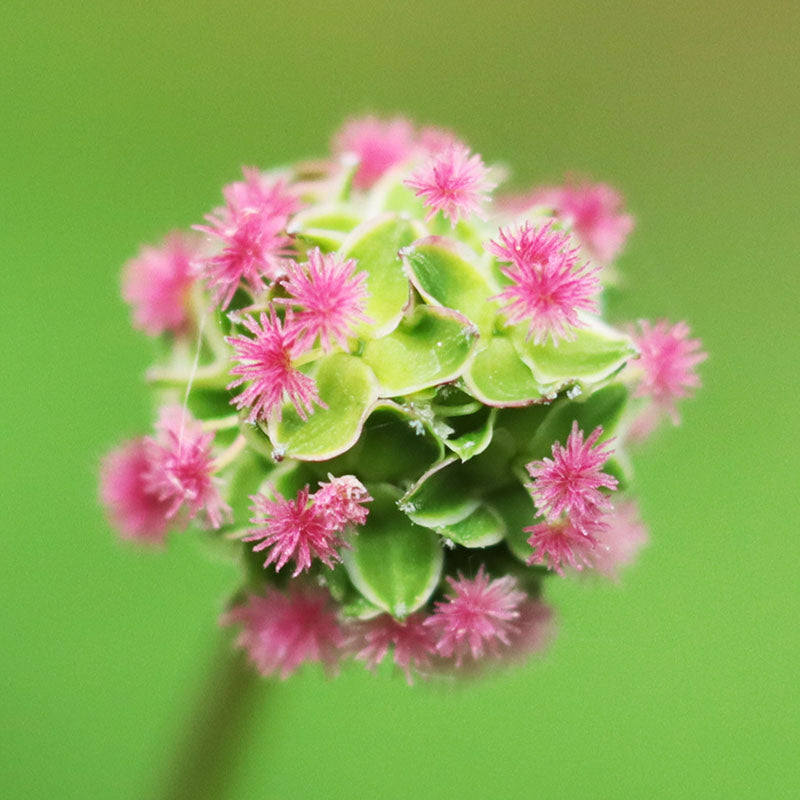In this vibrant photograph, we observe a flowering plant set against a bright, fluorescent green backdrop. The background is primarily lime green, with a patch of reddish-brown in the top right corner. The plant is centrally positioned, with its oval-shaped green leaves displaying white edges and a slightly stiff, pointed appearance. These leaves create a layered, bunched-up formation around the plant. Emerging from the ends of the leaves are numerous light pink flowers, approximately 25 or more. Each flower features narrow, elongated petals that darken towards the center bud, giving a prickly and almost intimidating look. The photograph captures the plant's exquisite contrast of colors—bright green foliage and vibrant pink blossoms—highlighted with varying degrees of sharpness; the center is in clear focus while the edges blur gradually.